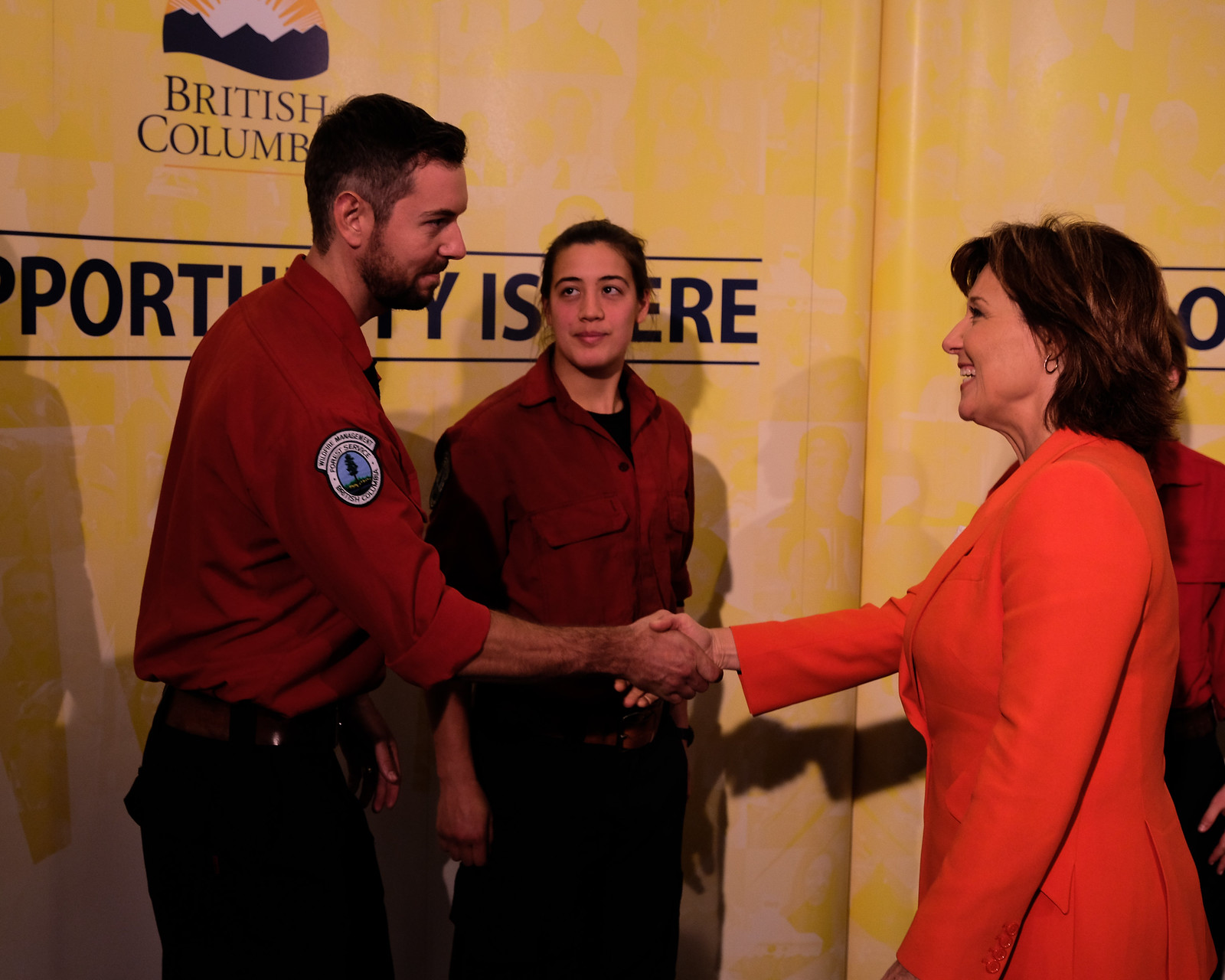In this photograph, we observe a detailed scene featuring four individuals. At the forefront on the right side, a woman with dark shoulder-length hair, light skin, and dressed in a formal, red-orange suit smiles broadly, her mouth slightly open, and extends her right hand to shake hands with a man. This man, taller and appearing to be a medical or forest service worker, dons a long-sleeved red shirt—rolled up to his elbows—with a logo featuring a tree on the right shoulder, dark pants secured with a white-brown belt, and possesses a mustache. Both individuals are engaged in a handshake, with their right arms extended toward each other.

To the man's left, partially in front of him, stands a younger woman. She faces the camera directly, wearing a buttoned, collared red shirt with a visible flap pocket on the front, and black pants with a black belt. Her dark hair is tucked behind her ears, and her eyes are fixed on the man, indicative of focus and attentiveness. 

In the background, to the left of the frame, there is another individual, mostly obscured by the woman in the red-orange suit, and clad in a similar uniform to the other employees, suggesting they may also be part of the same organization.

The backdrop features a wall with the British Columbia logo in yellow and white, accompanied by black lettering that reads "British Columbia" and larger text beneath it declaring "Opportunity is here," although some of the lettering is obscured by the standing figures. The lighting casts distinct shadows of the people against the yellowish wall, adding depth to the indoor scene.